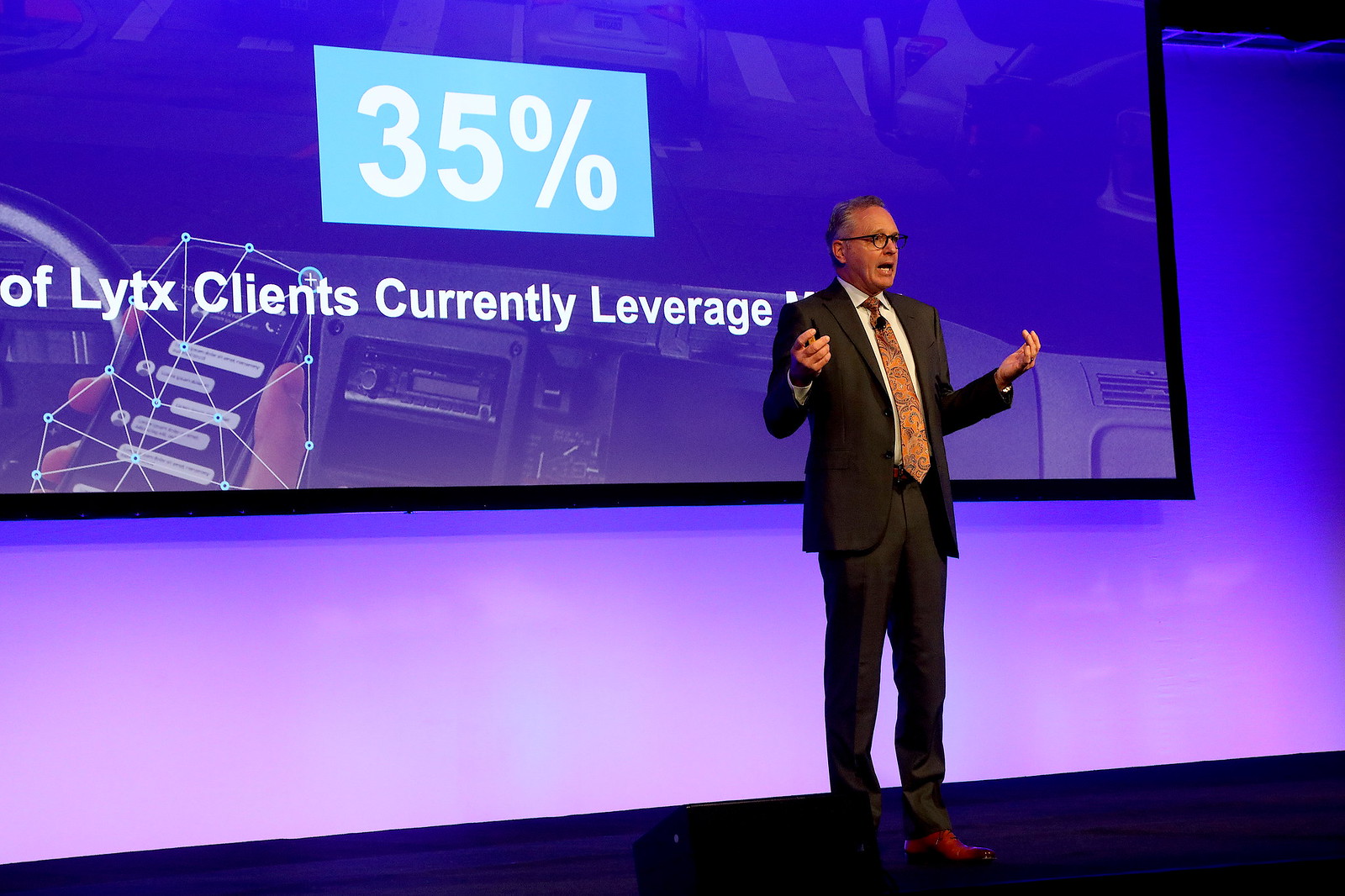A gray-haired Caucasian gentleman is giving a presentation on a dimly lit stage, creating a cozy and introspective mood. He stands off to the right of the frame, speaking energetically with both arms raised and hands cupped in a beseeching gesture. His sophisticated attire includes a black business suit, brown leather shoes, and a tan tie, complemented by a small microphone attached to his tie and spectacles. The backdrop is a gradient from light purple to dark blue, with a projector screen displaying large white text reading "35% of Lytx clients currently leverage" in an aqua blue rectangle. Both the stage floor and background are various shades of blue, tying the scene together in a cobalt palette. The photograph appears to be taken from the perspective of an audience member, capturing the action and atmosphere of a live indoor presentation.